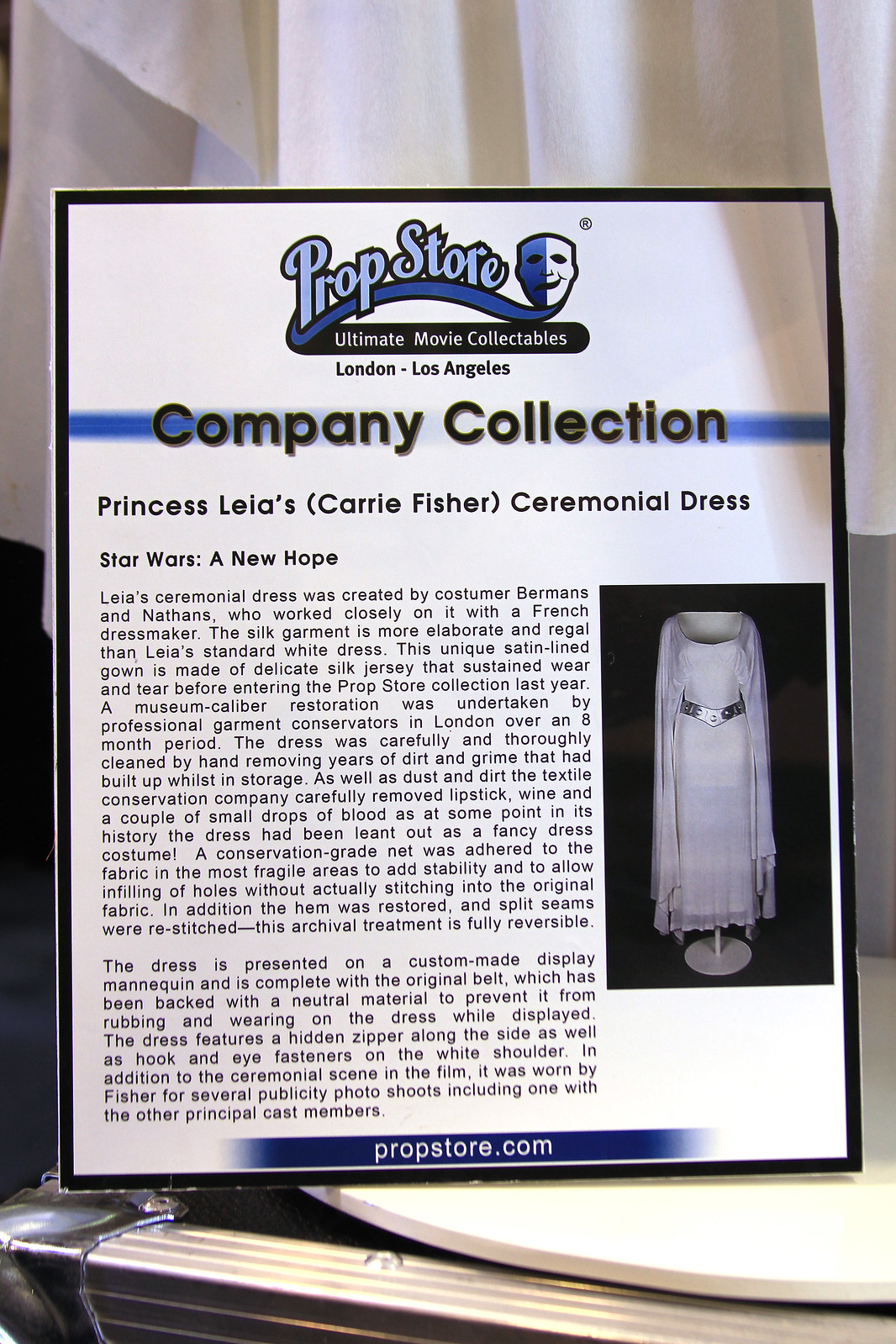This indoor photograph, taken in portrait orientation, showcases a detailed display marquis outlining Princess Leia's (Carrie Fisher) ceremonial dress from *Star Wars: A New Hope*. The marquis, bordered in black, features a header in blue and white that reads "Prop Store Ultimate Movie Collectibles," highlighting the company's London and Los Angeles locations. Beneath a horizontal blue strip with the text "Company Collection" in bold, it announces "Princess Leia's (Carrie Fisher) Ceremonial Dress," accompanied by a narrative and a photograph of the iconic gown. The dress, designed by Berman's and Nathan's collaborating with a French dressmaker, is a satin-lined, delicate silk jersey garment that underwent an extensive, eight-month museum-caliber restoration by London-based garment conservators last year. This process involved meticulous hand-cleaning to remove accumulated dirt, grime, and stains like lipstick, wine, and blood from its history as a fancy dress costume. Fragile areas were reinforced with conservation-grade netting, and the hem and split seams were expertly restored. Mounted on a custom-made display mannequin and accompanied by its original belt backed with a neutral material for preservation, the dress features a hidden side zipper and a shoulder hook and eye fastener. It was worn not only in the ceremonial scene of the film but also in several promotional photo shoots with the principal cast. 

Below the descriptive text, "PropStore.com" is displayed, and to the right, a full image of the dress on a black-backgrounded mannequin complements the narrative. In the background of the primary image, a portion of the actual dress and the lower part of its display mannequin are visible, linking the marquis with the displayed artifact.